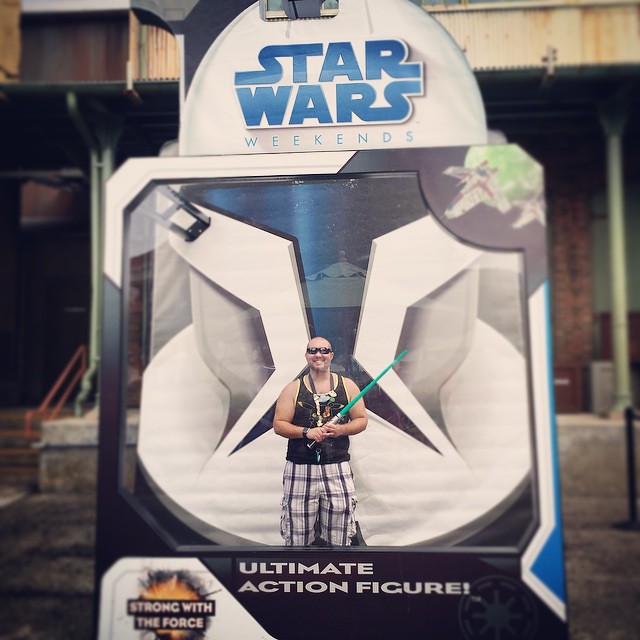This square image captures a man posing at a Star Wars exhibit within an amusement park, solidifying the theme "Star Wars Weekends" announced in bold blue font at the top. The backdrop features a giant, white, helmet-like figure emblematic of a Stormtrooper or Clone Trooper, adding a surreal ambiance to the scene. The man, who appears to be in his early 30s and is bald with a beard, stands confidently in the center of the frame. He is dressed in a black tank top with a graphic design and plaid shorts, complemented by sunglasses that reflect his cheerful demeanor. His attire includes accessories like a vibrant green lightsaber, which he holds prominently in front of his body, angling slightly to his top right. The entire photograph is encapsulated within a dark blue and silver border, akin to collectible card packaging, featuring additional text at the bottom in white stating "Ultimate Action Figure!" and "Strong with the Force." The background reveals a blurry, light-green metal scaffolding structure and several gray paved areas, adding depth to the lively atmosphere of the Star Wars-themed event.